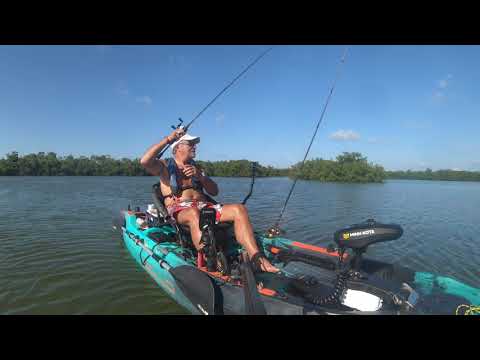In the image, an older gentleman is fishing from a turquoise motorboat, likely on a pond or lake with darker-colored water. He is dressed in flowered swim trunks, a white hat, glasses, and a life preserver, but no t-shirt or shoes. A black strap, likely part of the seat, stretches across his chest. He holds a fishing pole, while another pole rests in a holder attached to the boat. The boat also has a visible motor with coils and wires, and an oar attached to its side. The backdrop features dense green foliage and some small islands under a clear blue sky with a few scattered clouds.